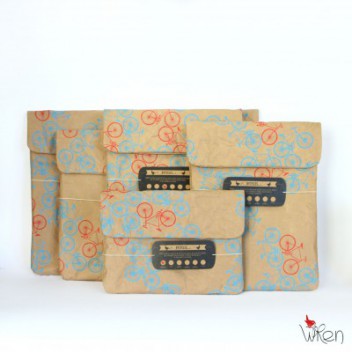This image is a product display from REN featuring a collection of five pouches designed for laptops or iPads. The pouches are standing vertically against a white background, which casts a slight shadow to the right. The pouches come in a pale peach or tan color, adorned with a whimsical pattern of light blue and occasional red cartoon bicycles facing various directions. The collection includes one small horizontal pouch in the front and four slightly overlapping vertical pouches at the back, each varying slightly in height. The pouches feature a flap or seal on top and an elastic band with a tag that has red dots, likely indicating the product size. Positioned in the lower right-hand corner, the REN logo appears with the letters "WREN" in thin black text and a small red cardinal perched on the W, adding a charming touch to the minimalist design.